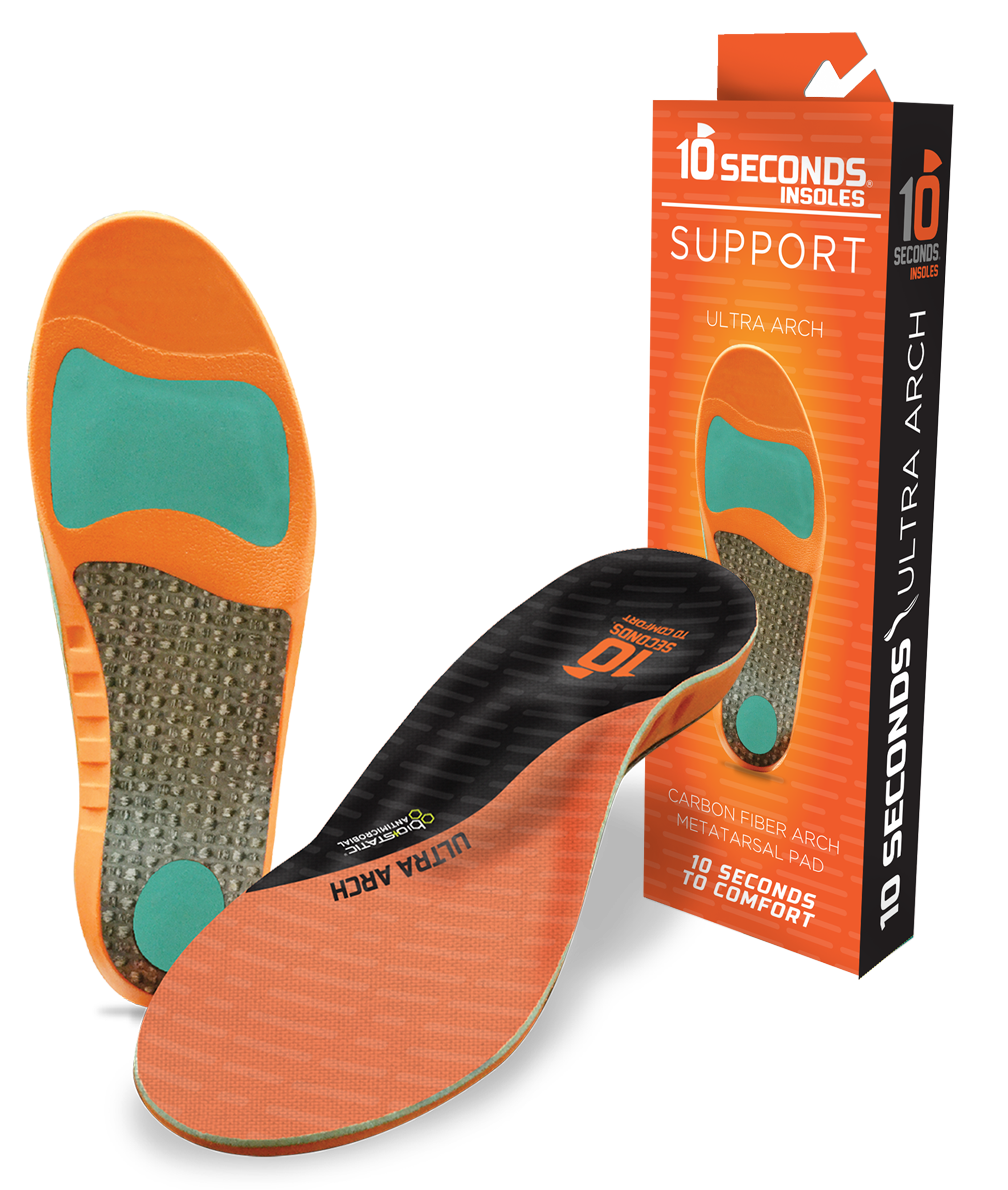This detailed photograph, likely intended for marketing or advertisement purposes, showcases a pair of orange insoles along with their product packaging. The image features two different angles of the insoles, highlighting their design. The insoles are predominantly orange with the top displaying a black and orange color scheme. The bottom of the insoles includes a grippy gray surface, with distinct cushioning sections: blue cushioning near the bottom, green cushions under the heel, and beneath the arch of the foot.

The insoles' packaging is also prominently featured in the photograph. The box is orange and black and contains the branding details in white text. The front and side of the box are labeled with "10 Seconds Insoles Support Ultra Arch," along with additional descriptors such as "carbon fiber arch" and "metatarsal 10 seconds to comfort." The packaging design includes very faint gray lines and the company's logos, with the number "10" stylized—the one in white or gray, and the zero in orange. The entire setup is captured against a white background, accentuating the product's vibrant colors and details often seen in professional marketing images.